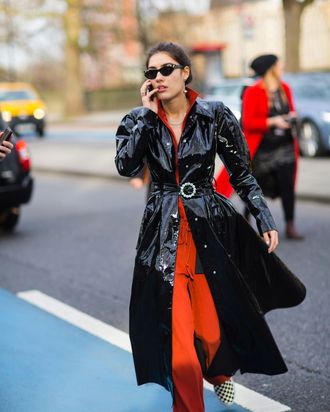In this image, a trendy Caucasian woman is walking towards the camera while talking on her cell phone. She is wearing dark sunglasses and a shiny, black leather-like trench coat, which is buttoned in the front and belted with a large, possibly diamond-studded silver buckle. Her brown hair is tied back, possibly in a ponytail, keeping it off her face. Under the trench coat, she is donned in an orange or red outfit, either a suit or a jumpsuit. Completing her ensemble are black and white checkered slip-on shoes. She is crossing a street, with a few cars—black, yellow, and bluish-gray—in the background. Also visible behind her is another woman dressed similarly in a long red coat over dark clothing and a dark hat, with blonde hair. Both women are in motion, contributing to the dynamic urban scene.